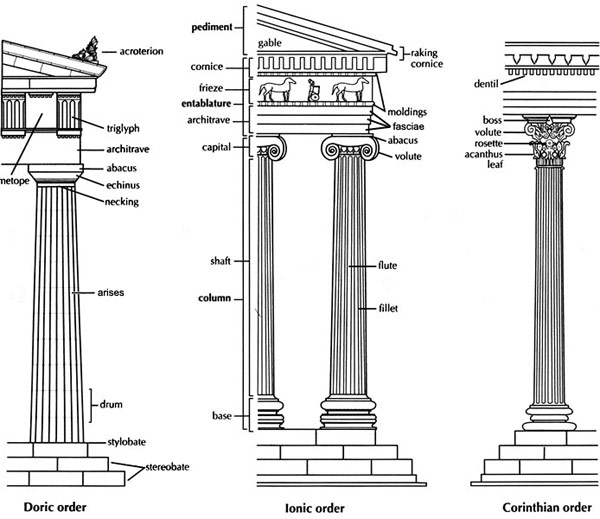The black ink drawing on a white surface is a meticulously detailed graphic illustrating the three classical orders of Greek columns: Doric, Ionic, and Corinthian. Each column is richly annotated, highlighting the intricate components that comprise their structures.

On the left, the Doric order is depicted with about ten distinct elements identified, including fundamental parts such as the top section (called the entablature) and the base. This diagram points out specific features like the triglyph, and necking, making it clear that this architectural style is characterized by simplicity and strength.

In the middle, the Ionic order, known for its elegance and scroll-like volutes, includes a more extensive list of approximately fifteen elements. The diagram showcases components such as the raking cornice, pediment, frieze, and entablature. These annotations reveal the complexity and level of detail that define the Ionic style, with attention to intricate moldings and sculptural details on the columns.

On the right, the Corinthian order is represented, albeit with fewer annotations—only about five components are labeled. This column style is distinguished by its elaborate capital adorned with acanthus leaves and a rosette. The limited number of labels suggests that some features, like the fluted shaft with its fillets, are shared with the other column styles and perhaps only uniquely intricate details are highlighted here.

Overall, the drawing serves as an in-depth instructional guide, illustrating the fundamental architectural elements of classical Greek columns with clarity and precision, emphasizing both the commonalities and unique traits of each order.